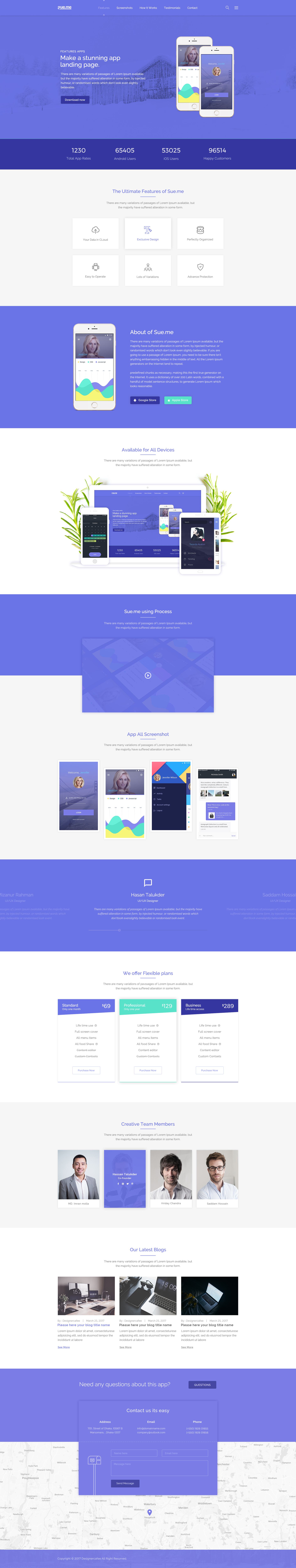The image captured from a cell phone screen showcases a well-designed landing page for an app called "su.me." At the very top of the page, prominently displayed text reads "Make a Stunning App Landing Page," followed by sections titled "About su.me" and "The Ultimate Features of su.me," which detail six key features. 

The layout of the page alternates between dark periwinkle and gray sections, creating a visually appealing contrast that guides the viewer's eye downward. In one of the central sections, an iPad is depicted, presumably showcasing the app's interface.

Toward the bottom of the page, there are images of three men identified as "Creative Team Members," with their names listed below their photographs. Adjacent to this, a section titled "Our Latest Blogs" provides clickable links to three recent blog posts.

Finally, at the very bottom of the page, a subtle map in fine print is visible just beneath a section labeled "Contact Us," which offers assistance and answers to potential questions about the app.